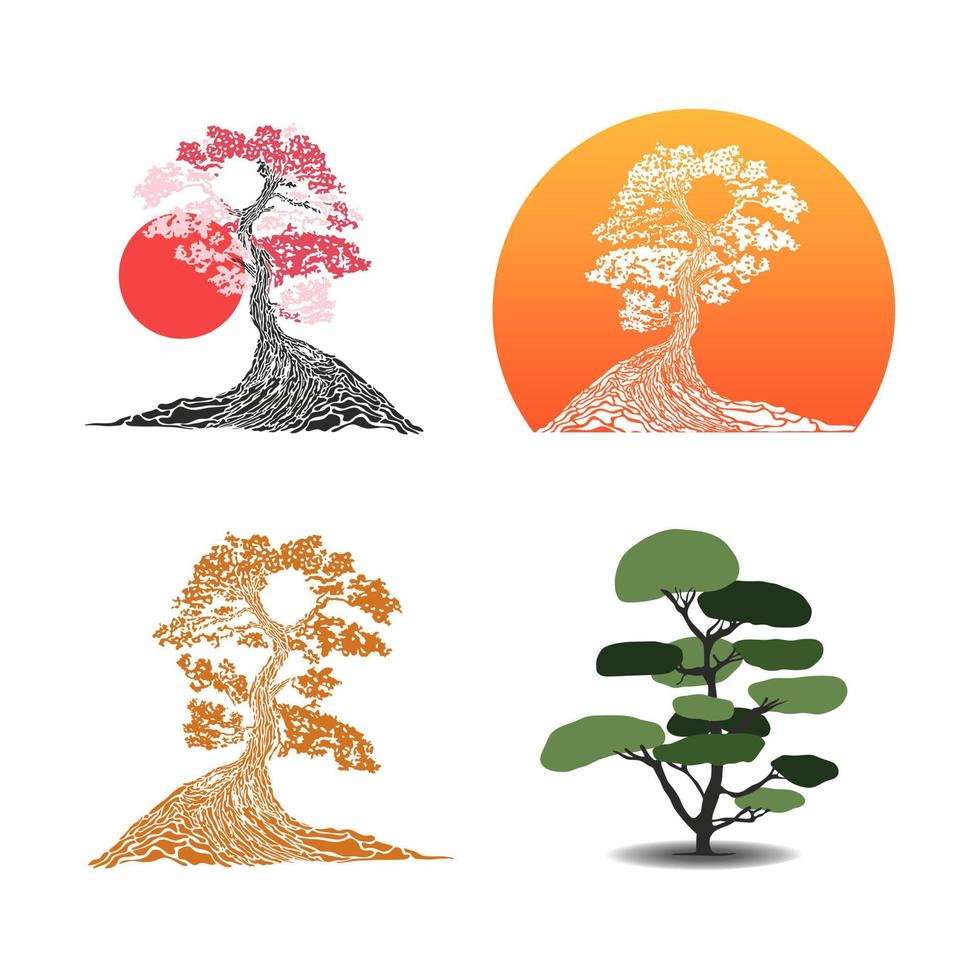The image features four distinct digital illustrations of Asian-style trees, each occupying one corner. In the top left corner, there's a tree with thick roots and branches adorned with dark and light pink leaves, set against a red, sun-like circle background. The top right corner mirrors this tree but in stark white, set against a gradient orange sun that darkens towards the bottom. The bottom left corner showcases a similar tree rendered in shades of orange. Finally, the bottom right corner presents a bonsai-like tree with varying shades of green blobs representing leaves, branching out from a central black trunk.